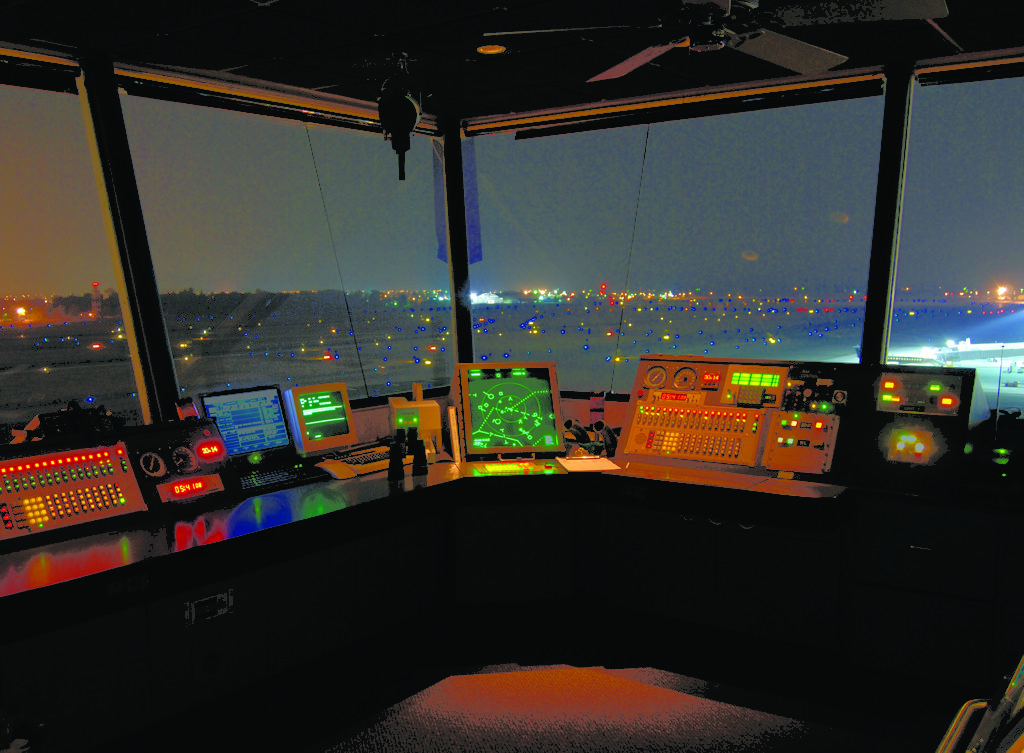This night-time image captures the interior of an airport control tower, specifically the ATC (Air Traffic Control) office. The scene offers a panoramic view of the dimly-lit room, illuminated by an array of vibrant colored lights, including blue, yellow, red, and predominantly green, which reflect off surfaces, adding a vivid contrast to the setting's darkness. The room is enclosed by large glass windows, providing a view of the brightly lit runway and night sky beyond. Inside, a black ceiling features a fan, contributing to the room's functional yet subdued ambiance.

The control tower's workspace is dominated by a long desk that runs along the windows, cluttered with a variety of specialized equipment. Numerous monitors display maps and other critical information, and are accompanied by lit-up buttons and control panels that emit an assortment of colors. A chair is positioned in front of this sophisticated control interface, which also includes binoculars, keyboards, and other essential operatives' tools. The reflective surface of the desk and the assortment of illuminated controls enhance the complexity and high-tech nature of this vital airport facility.